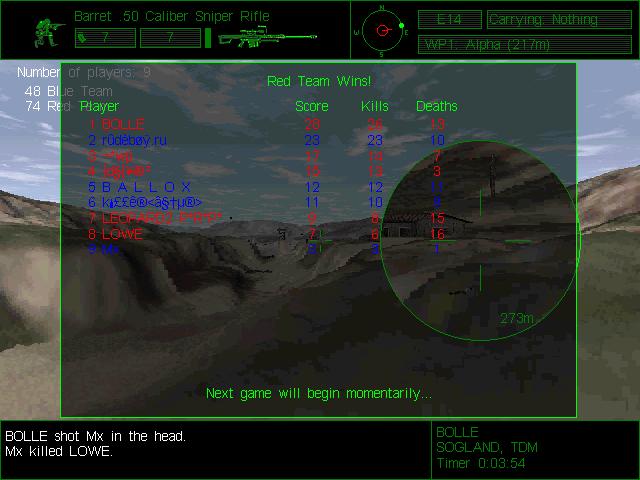In the freeze-frame of the video game, a vast desert terrain stretches out below, its arid landscape dissected by a dry ravine. The screen is overlaid with detailed data in red and blue, indicating the scores of kills and deaths for each team. The match has concluded with the declaration "Red Team Wins" prominently displayed, indicating the victorious team. A countdown informs players that the next game will commence shortly. On the right side of the screen, a circular target indicator with telescopic lines marks the player's aim. At the top, a soldier clad in army gear is visible, wielding a rifle. The display includes the text "Bally shot in the head" along with the identity of the player who made the kill, providing comprehensive details about the gameplay action.